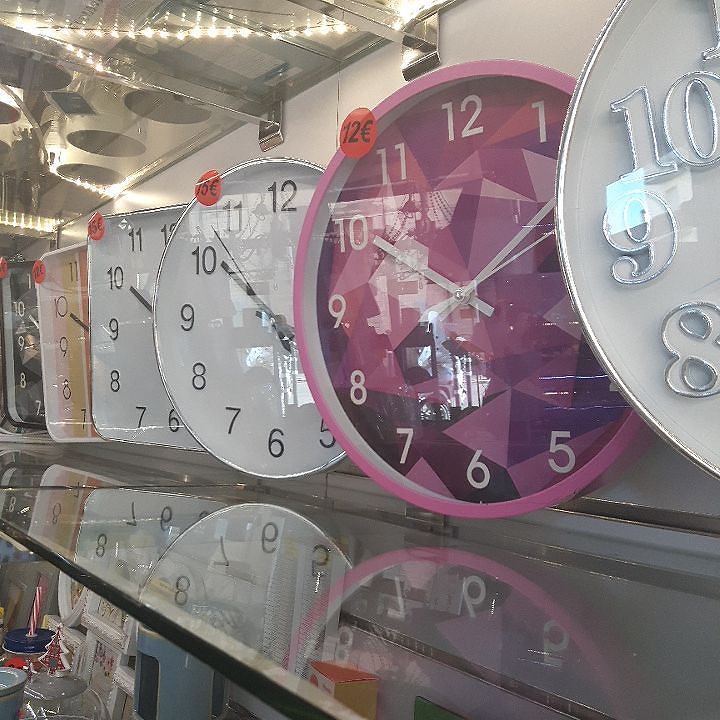The image is a color photograph taken inside a store, possibly through a window or glass case, showcasing a glass shelf with numerous wall clocks. The shelf itself has a metal frame and edge, but the main part is glass, reflecting the clocks above it and creating a mirrored effect. There are six visible wall clocks, comprising both round and square shapes. Starting from the right, there's a white clock with silver-edged white numerals and a silver frame. Next is a round clock with a pink frame featuring various shades of pink and purple geometric shapes, white numerals and hands, and a sticker indicating its price at 12 euros. The subsequent clock has a white face with a silver frame and numerals, priced at 15 euros. Further left are several square-shaped clocks with white faces and different colored details including tan, orange, and black. All clocks appear to be battery-operated and indicate roughly the same time, around 10:10. Below this glass shelf, partially visible in the bottom left corner, is another glass shelf holding what seems to be candles or glasses. Reflections from the glass surfaces and clock faces add a layer of complexity to the scene.